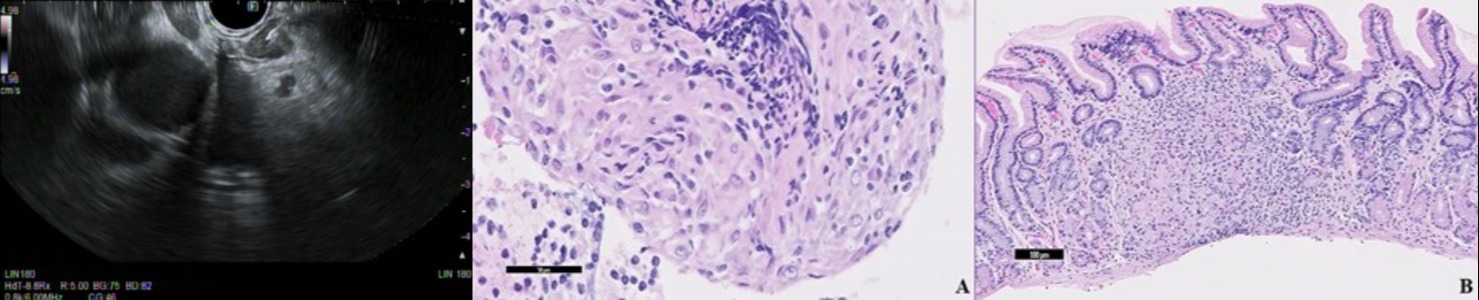The overall image is a horizontally aligned rectangular collage composed of three separate horizontally rectangular images. The image on the far left is a predominantly black and white scan, resembling an ultrasound. It features dark gray masses and faint light gray areas, forming a half-circle shape typical of a sonographic view. The center image is shaded in light and dark purples, showcasing a large, rounded center with clusters of darker purple speckles scattered throughout a lighter purple background, encircled by white. The far right image, also primarily purple, depicts a curved rectangular shape with branching, flame-like extensions emanating from the top. It is outlined in a deeper purple hue with numerous tiny speckles scattered within a lighter purple interior, surrounded by either white or light gray. Text is minimal and appears in black, with "A" labeling the center image and "B" labeling the right image. The content appears to be microscopic views of cells or nerves, but the exact identification is unclear.